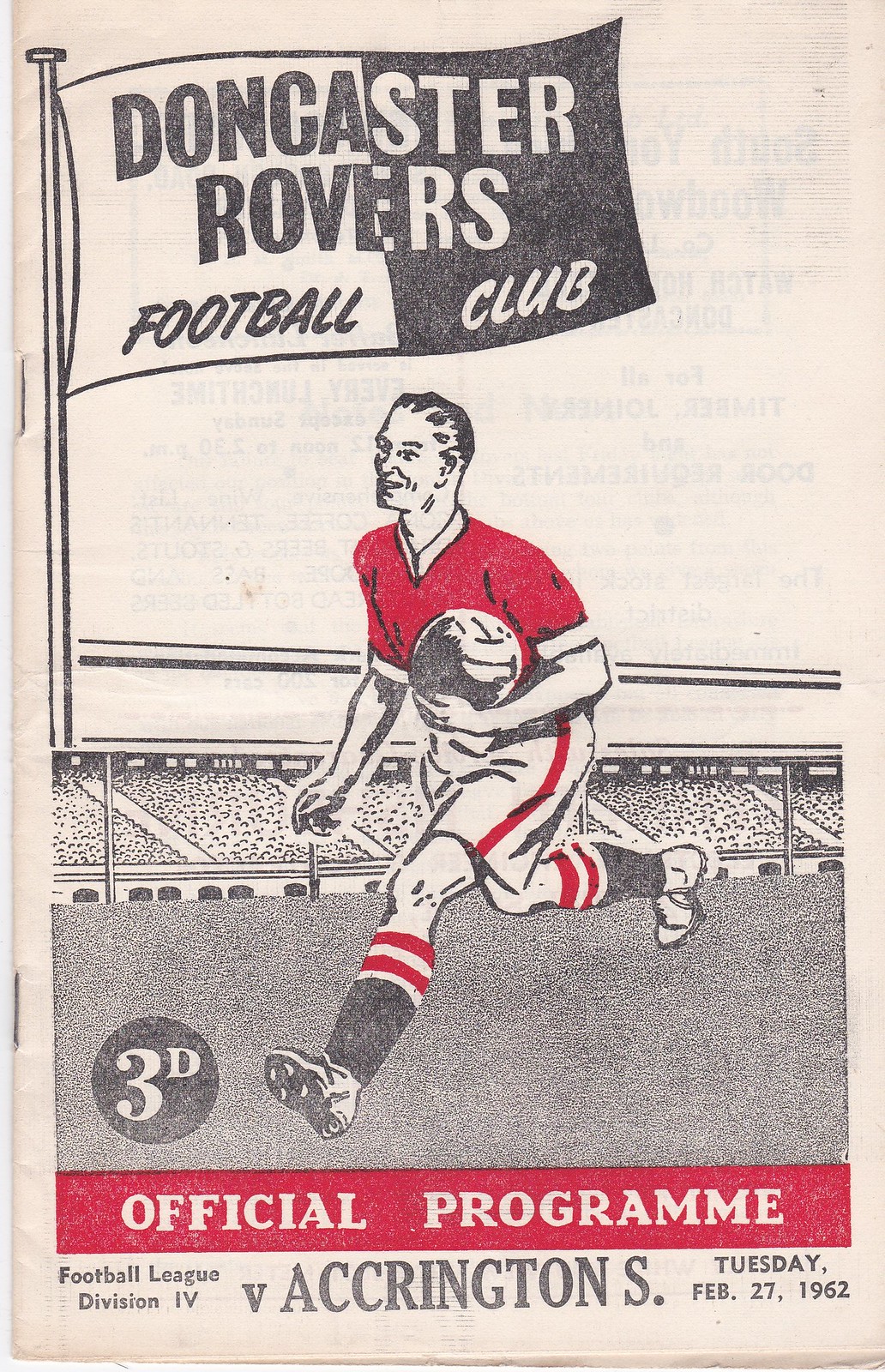The cover image of the game day program showcases a detailed illustration in black, white, and red. Dominating the scene is a cartoon soccer player wearing a red shirt with red stripes and white pants, complemented by black socks with red and white striped tops. He is captured mid-run, clutching the ball under his arm, against an indistinct background suggesting a stadium filled with spectators, represented as tiny dots. On the left-hand side of the illustration, a tall flagpole carries a flag emblazoned with "Doncaster Rovers Football Club," with the text split into black on a white background and white on a black background. Additionally, a small circle near the player's foot features the text "3D." At the bottom of the cover, a red horizontal bar with white lettering designates it as the "Official Program." Below this, in black text, the details read: "Football League Division IV vs. Accrington S., Tuesday, February 27, 1962."